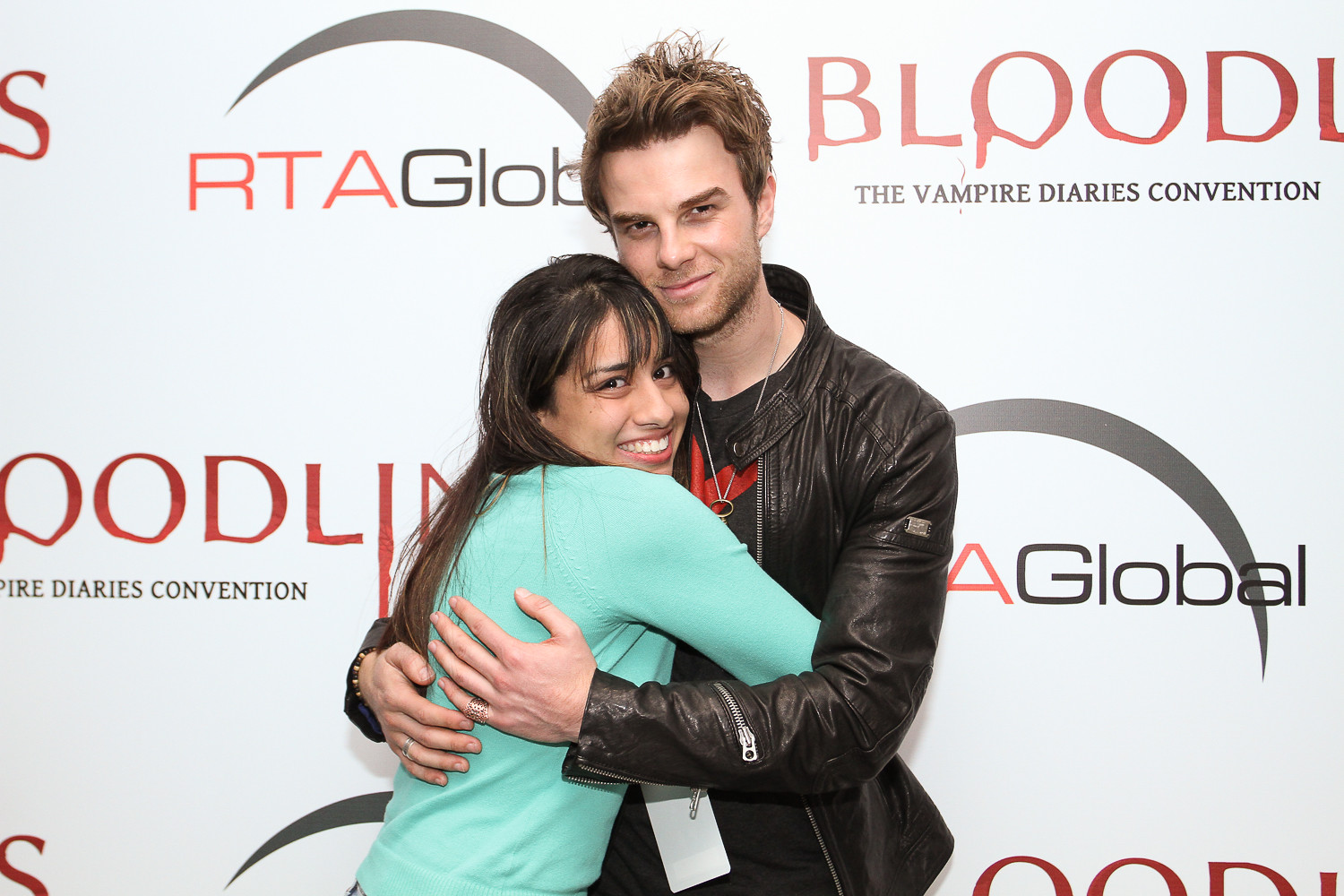This photograph captures a heartfelt moment at The Vampire Diaries Convention, depicting an actor and a fan embracing against a promotional backdrop. The young man, positioned on the right, sports a black leather jacket over a black t-shirt with a red graphic, and he has light brown, slightly tussled hair and a bit of stubble. Around his neck hangs an unidentifiable name card. The fan, nestled into his embrace, wears an aqua green sweater, has long dark brown hair with bangs, and displays a radiant smile, clearly thrilled by the encounter. Both appear to be in their 20s or 30s and are looking directly at the camera. Behind them, a white backdrop features repeating logos: one with a gray upward crescent and "RTA Global" in red and gray letters, and another with "Blood" in red drippy letters and "The Vampire Diaries Convention" in black serif font. The overall scene beautifully captures the fan's excitement and the warm interaction with the actor, set against the characteristic promotional wall of such events.